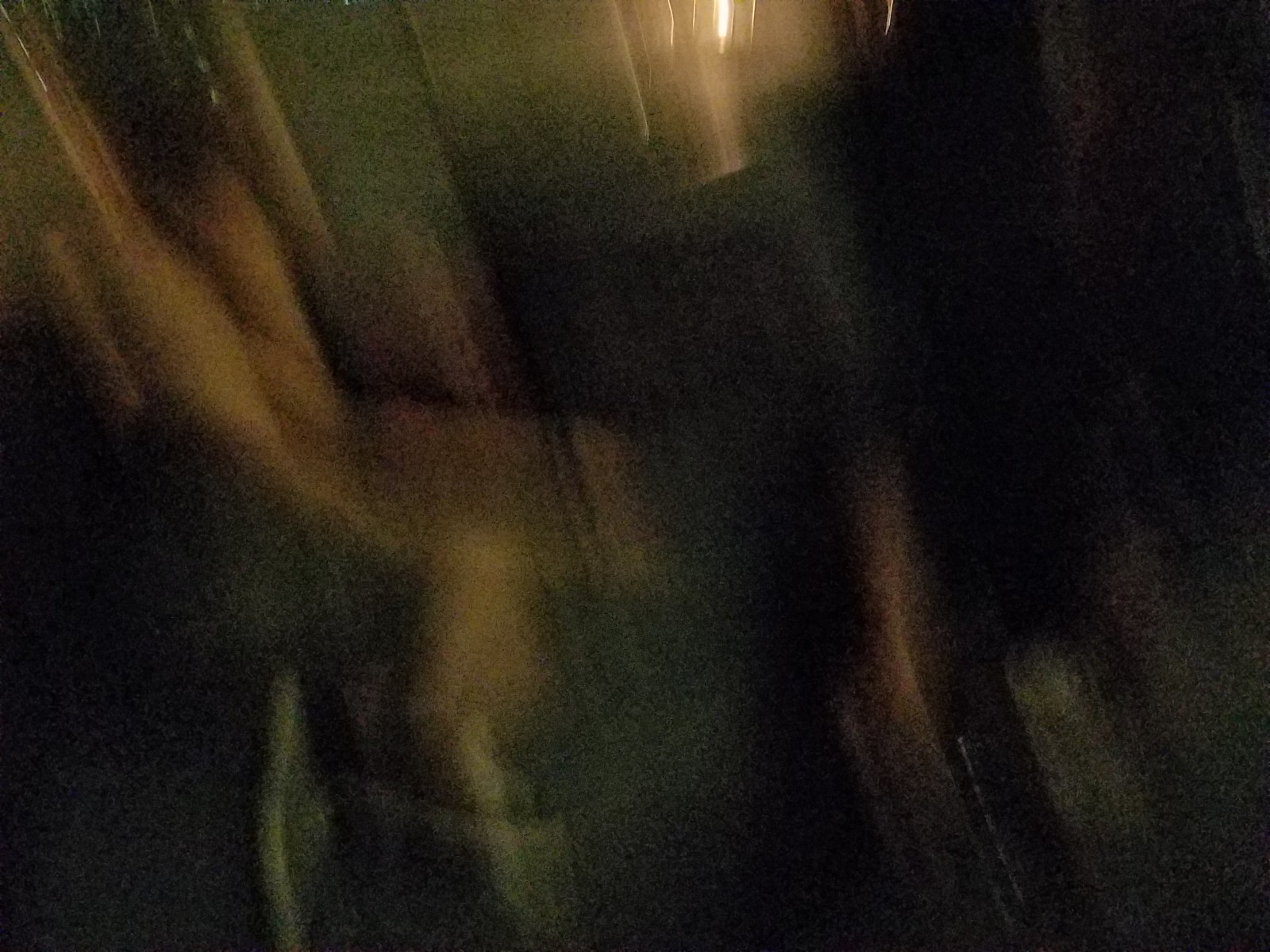This color photograph, taken in low-light conditions, is extremely blurry, dominated by streaks of darkness and muddled movement, resulting in an abstract composition. Prominently, at the top center of the image, a golden light forms a focal point with radiant lines suggesting motion, potentially indicating headlights or a similar bright source. The overall scene is so unclear that it is difficult to discern the exact setting; possibilities include the interior of a room or the view from inside a moving vehicle. The left side of the photograph features a streak of golden yellow light, adding to the ambiguity. Despite the murky gray and green tones enveloping the scene, the photograph retains an indistinct, ghostly presence of shapes, with some areas hinting at the outline of bottles or other objects.